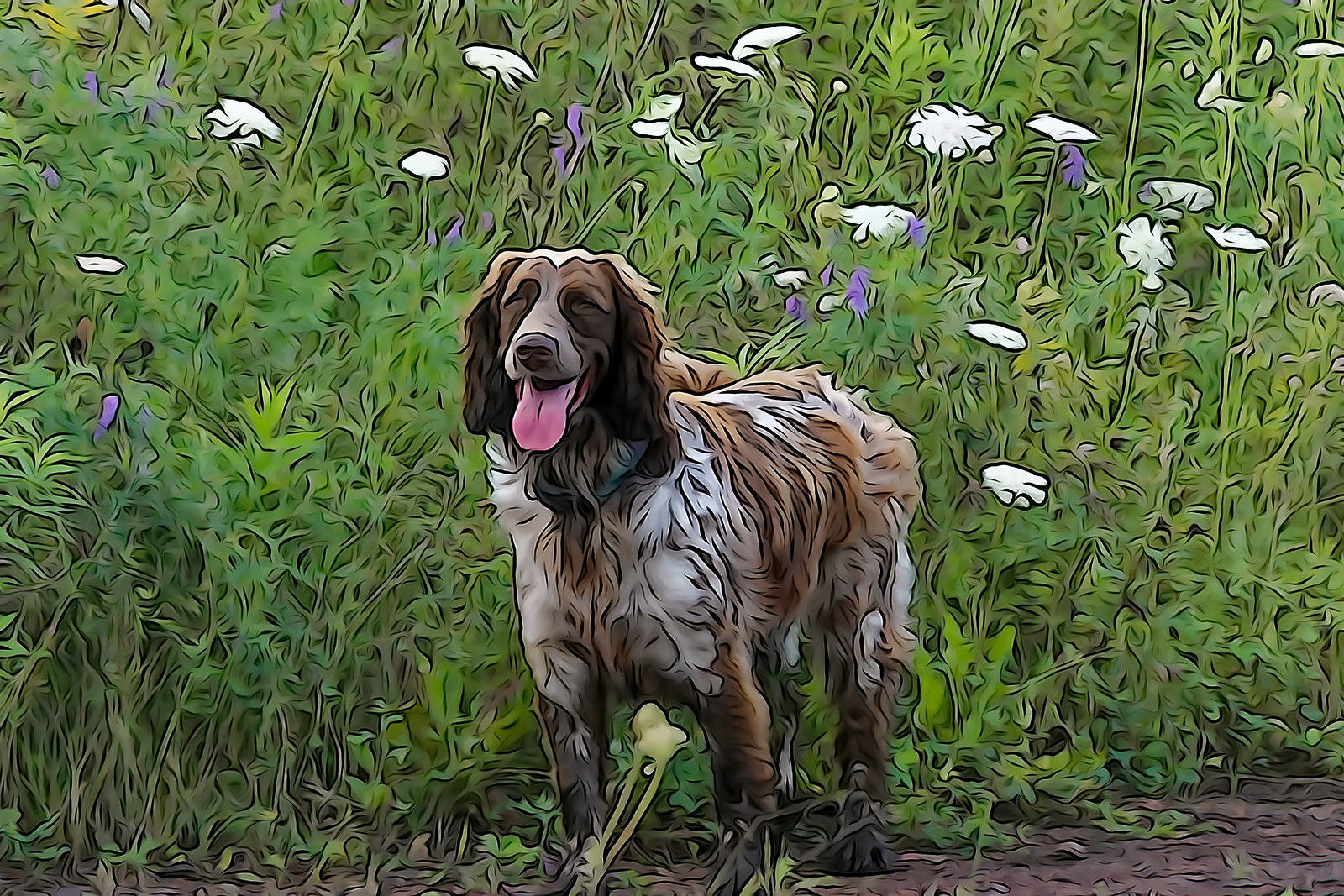This image features an artistic rendering of what may have once been a photograph, transformed with a psychedelic animation overlay into a detailed and vibrant cartoon watercolor. The focus is a large cocker spaniel mix or possibly an Australian shepherd, standing in the center on all four legs. The dog has its eyes closed and appears to be very happy, with its tongue sticking out and a smile on its face. 

The dog’s shaggy coat is a blend of white and light brown, with a darker coloration on its face and large floppy ears. It stands in a field of tall greenery, where the plants—including scattered white and lavender flowers—tower above it. The background is infused with fluorescent pink hues, adding to the psychedelic, drippy pixelation effect that blurs the definition of the overgrown weeds and flowers. The surface beneath the dog’s paws is an indistinct dirt path. This image merges the elements of a photograph and artistic animation to create a vivid, dream-like scene centered around the joyful dog.